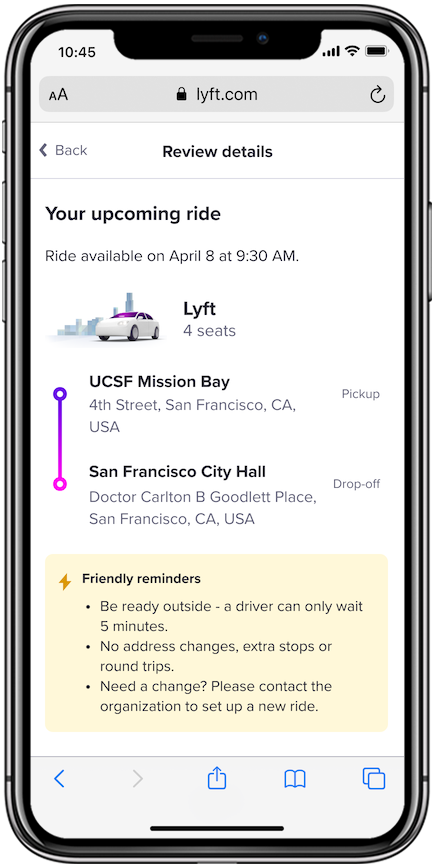The screenshot displays an iPhone interface with a white background. The status bar at the top shows the time as 10:45 in black text, with icons indicating battery life, cell signal strength, and WiFi signal strength on the right side. Below the status bar, there is a grey background with two capital "A" icons for adjusting text size on the left side—one smaller and one larger. Centered below is a padlock icon followed by the URL "lyft.com" spelled out as L-Y-F-T dot C-O-M. A refresh circle icon is positioned on the right side.

A horizontal line separates this section from the content below. Beneath the line, on the left side, there is a "Back" option with an arrow pointing left. The center of the screen prominently features the text "Review Details" in bold, capital letters. Further down, in larger font, it says "Your Upcoming Ride," with "Your" capitalized.

Below this header, the details of the ride are presented: "Ride available on April 8th at 9:30 AM," capitalizing the first letters of "Ride," "April," and the "AM." It is followed by "Lyft - 4 seats," alongside an image of a white car. The journey is detailed as "UCSF Mission Bay to San Francisco City Hall."

Towards the bottom of the screen, a yellow background contains friendly reminders: "Be ready outside, no address changes, extra stops or round trips. If you need a change, please contact the organization to set up a new ride."